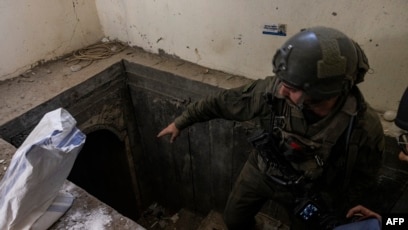The image depicts a man in military gear, characterized by a dark gray helmet and an olive full-body outfit, standing partially inside a rectangular cutout resembling a bunker or basement entryway in an old building. He is pointing down into the hole, suggesting he is either entering or exiting the space. The environment appears dirty and dusty, with cream-colored walls and visible signs of disrepair. To the left of the man, there is a white bag and some white powder scattered on the ground. An arched doorway is visible further inside the basement or bunker. In the lower right corner of the image, the text "AFP" is visible in white.